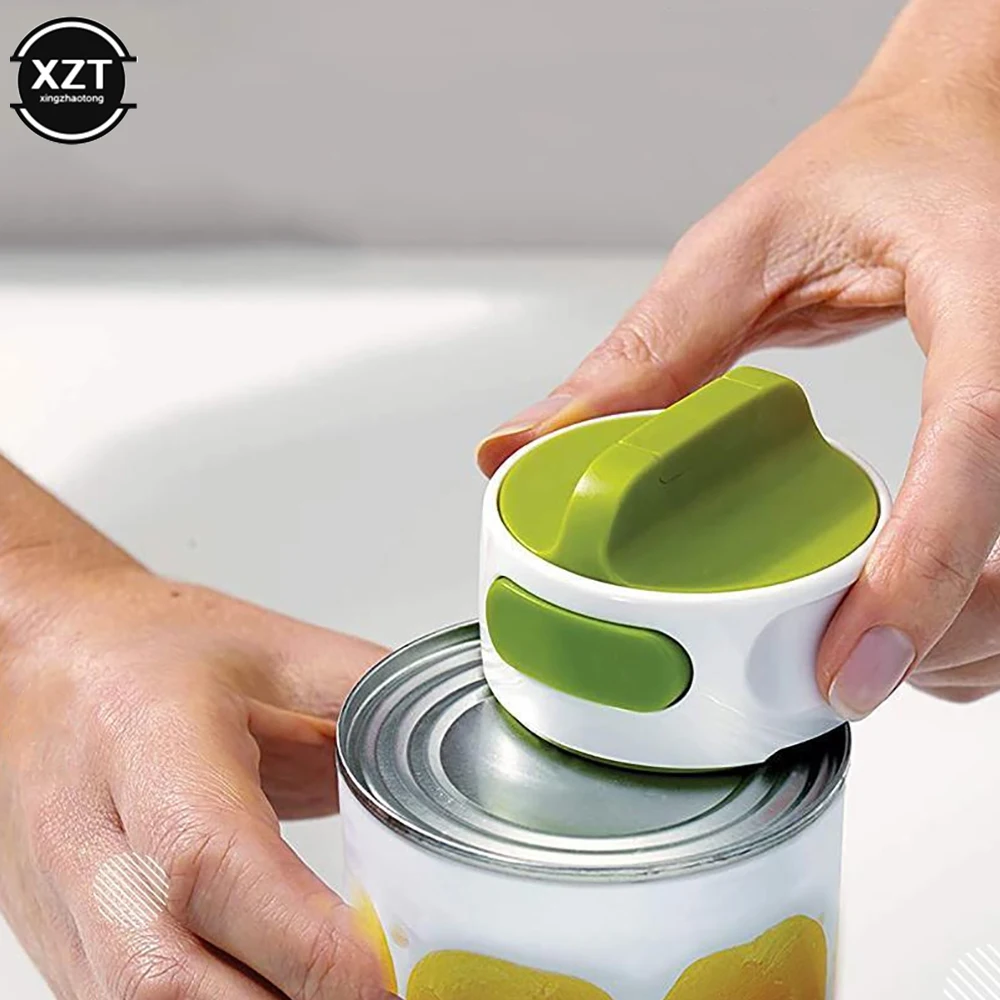This close-up, color photograph prominently features an innovative can opener in action. The device, which resembles a futuristic kitchen gadget, is a white disc approximately two to three inches tall, equipped with a green dial at the top that is similar to a kitchen timer. A small green button is also visible on the front of the device. The can opener is being used by two hands—one positioned at the top right of the image (holding the opener) and the other at the bottom left (steadying the can). The can, which has a white label adorned with orange and yellow designs, possibly depicting fruit, is being effortlessly opened by the sleek, white opener. In the top left corner of the photograph, there is a black circle containing the letters "XZT" in white, suggesting a brand logo. Below the logo, "XING ZHA OTONG" is clearly written, likely the name of the company. The overall composition and branding elements indicate that this photograph is likely an advertisement showcasing the ease and convenience of this electronic can opener.